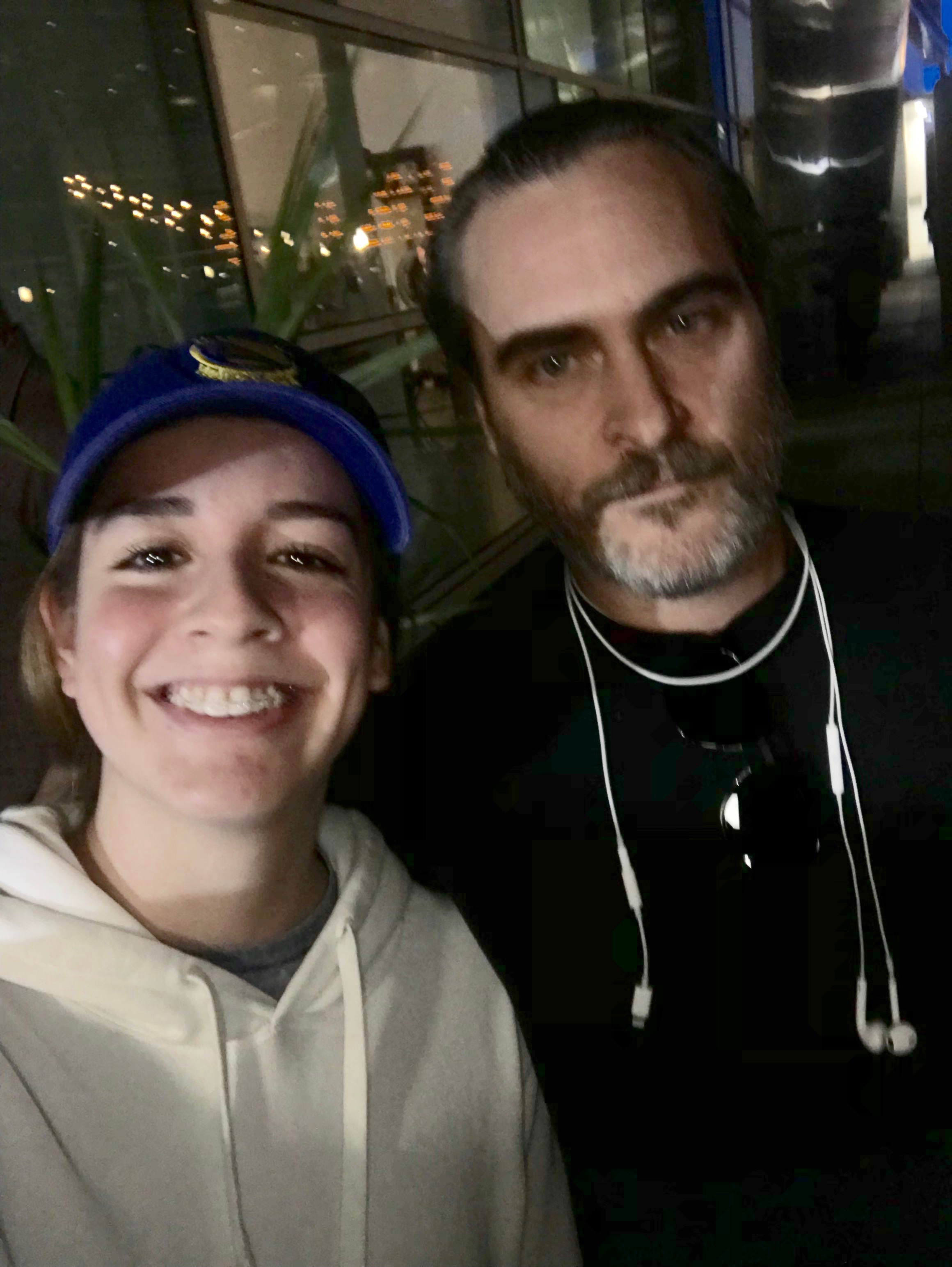In this detailed image, a young woman, likely in her early 20s, is taking a selfie with Joaquin Phoenix, the acclaimed actor. The woman, who has short brown hair and is smiling broadly to reveal her braces, wears a white hoodie over a gray shirt. She sports a dark blue-purple baseball cap adorned with a gold circular symbol at the center. Joaquin Phoenix stands to her left, appearing composed with his distinctive gray beard, dark mustache, and dark eyes, framed by dark eyebrows. He dons a black shirt with white Apple earbuds wrapped around his neck, their plug-in clearly visible. Both individuals are positioned outdoors in front of a series of glass windows, which reflect a cityscape with lights and buildings. Behind them, a partially open doorway illuminated with light and a green plant are also visible, adding depth to the lively urban background.